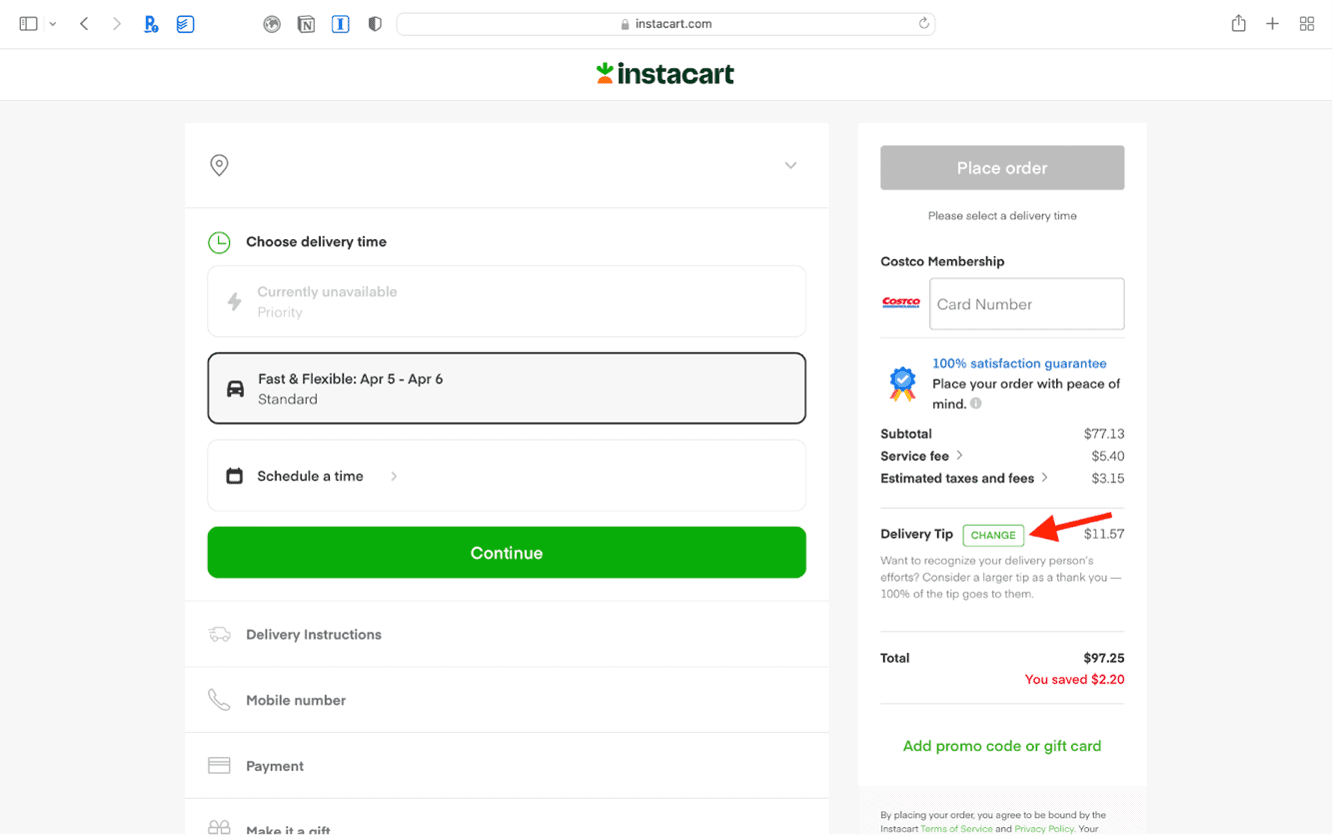This image captures the checkout portion of the Instacart website. Dominating the upper section is the Instacart logo, featuring the iconic carrot, centrally positioned. The screen primarily displays the "Choose Delivery Time" section. Under this section, the selectable option is "Fast & Flexible," with a delivery window spanning from April 5th to April 6th. Below these details are options to "Schedule" and "Schedule a Time," and beneath them, prominently, a "Continue" button.

On the right-hand side, a vertical menu is visible. Notably, the "Place Order" button is grayed out, indicating it's not currently clickable. Further down, there is a section labeled "Costco Membership," which prompts users to enter their membership number, highlighted with a red arrow for emphasis. Towards the bottom, the delivery tip section is shown with a green "Change" button, indicating that the tip amount can be adjusted.